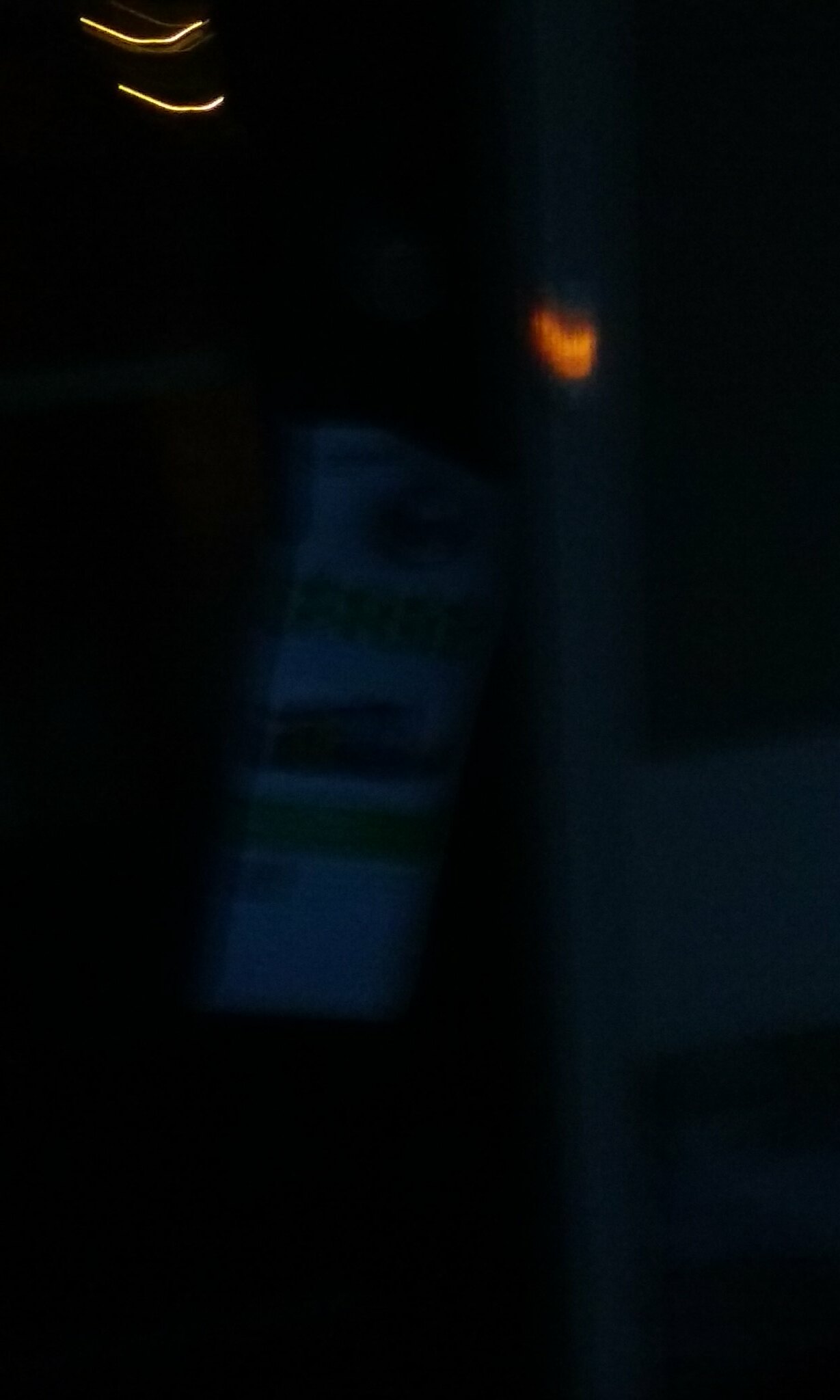A very blurry and dark image, predominantly in shades of black or charcoal gray. In the center, slightly off to the left of the vertical middle, there is an angled rectangle in a dark steel gray or bluish hue, featuring alternating strips of lighter and darker colors within it. Emerging from the right center of the image is another lighter colored area that ends in a vertical line. At the top of this vertical line is a small, curved amber light. In the upper left corner of the image, two parallel, partially curved yellow lines are visible, with the upper line dipping in the center.